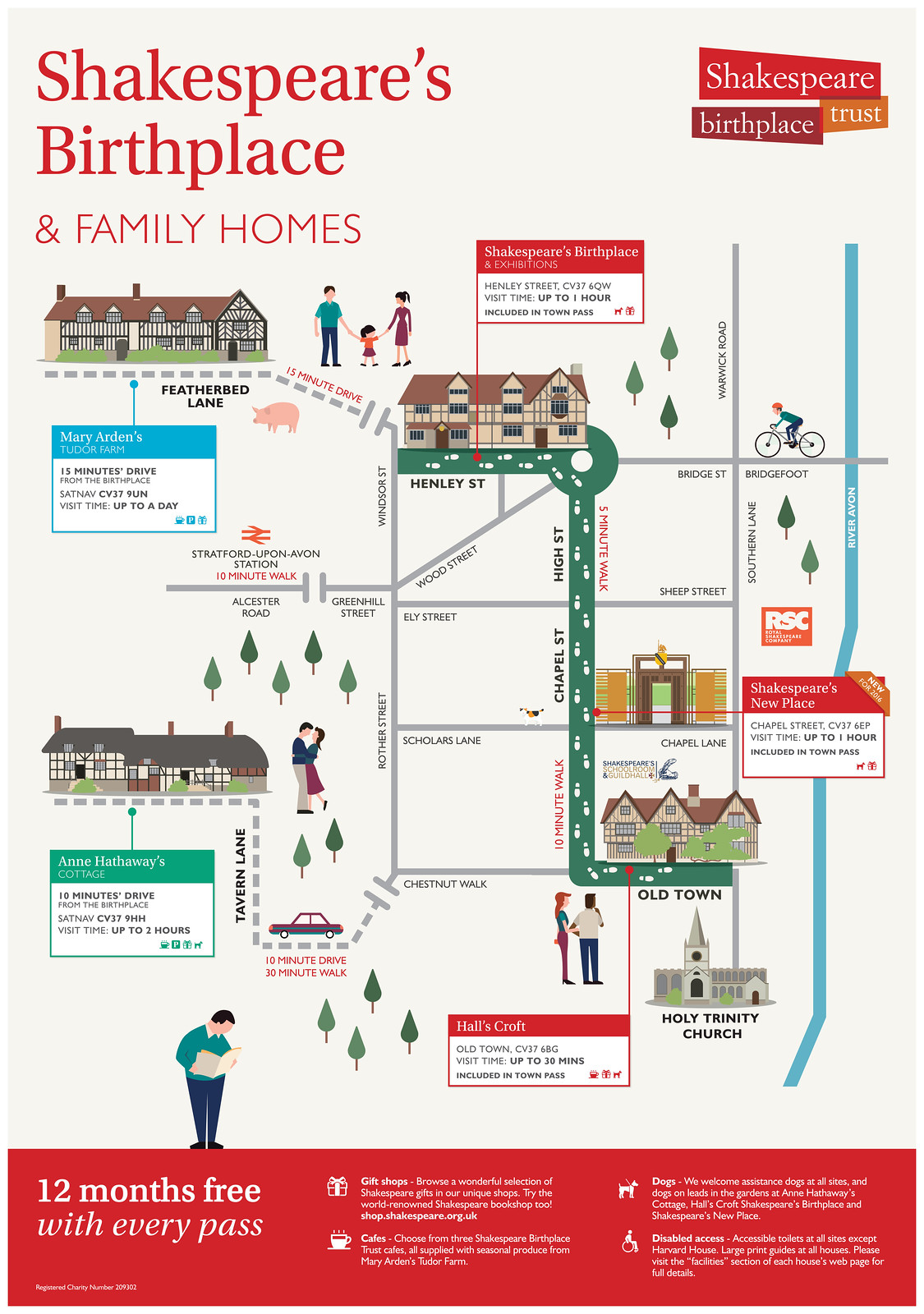The image is a poster designed to showcase various significant locations linked to Shakespeare's life, similar to a map. At the top, the headline "Shakespeare's Birthplace and Family Homes" can be seen, along with the logo of the Shakespeare Birthplace Trust. Below this, multiple illustrated depictions of different houses, roads, trees, and people are scattered throughout the poster. Key places are connected by colored lines and circles, resembling routes.

Details in the image include individuals cycling, a family with a man, woman, and child, a piggy bank, couples either standing and holding hands or kissing, a car, and a person holding a book. The routes and locations are labeled, with specific mentions like "Feather Lane," "Stratford upon Avon station," "Chestnut Walk," and "Shakespeare's Birthplace and Exhibitions."

At the bottom of the image, there is a prominent red rectangular strip with text stating "12 months free with every pass." Additionally, logos and text provide information about amenities such as gift shops with Shakespearean items, cafes using produce from Mary Arden's Tudor Farm, and facilities for disabled access. Details like a peace sign, a cup of tea, a dog, and a wheelchair highlight the user-friendly aspects of these locations. The poster features vibrant colors including tan, red, maroon, orange, green, yellow, brown, black, and blue.